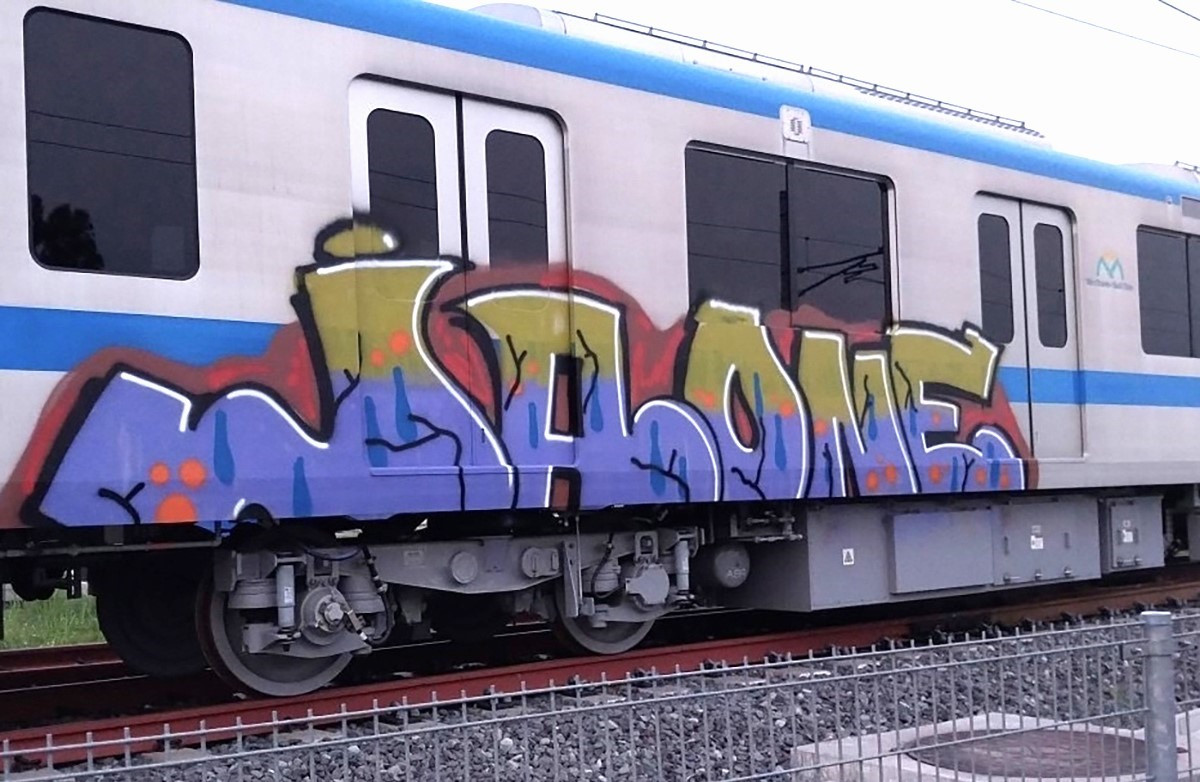Here we have a detailed photo of the side of a train, positioned on red steel tracks amidst an outdoor setting. The train, primarily composed of steel and metal, features a gray mechanical base and a blue roof. The side panel of the train is white, accented with a blue stripe running across its length. A prominent aspect of the image is the large piece of graffiti that spans almost the length of three doorways on the train's side. The graffiti, difficult to decipher but potentially spelling out “I-A-O-N-E,” showcases a blend of colors including olive green on the upper half and dark blue on the lower half, intertwined with black vein-like lines and surrounded by a dark red shadow. The scene is grounded by a metal fence, standing approximately three to four feet tall, and scattered rocks and gravel spread out below.